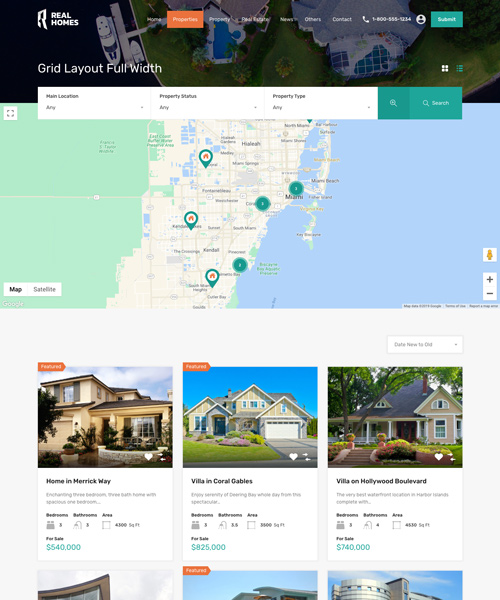The image depicts a real estate website with a header section featuring an aerial background image showing two houses perched near a pier wall edge with water extending beyond it. One house has a landing that stretches into the water with a larger boat docked there, while a smaller boat is visible at the upper left of the header.

In the upper left corner of the header, there's a logo followed by the text "Real Homes." To the right, the navigation menu includes several options with the "Home" tab highlighted in orange. Other menu items include "Properties," another unreadable option likely "Real Estate News" due to low image resolution, followed by "Contact," which features a phone icon and a 1-800 number. There's also a silhouette of a person and a blue "Submit" button with white text.

Below the header, there is a filtering section where users can select options such as "Main Location," "Property Status," and "Property Type." To the right of these filters are two magnifying glass icons, the first with a "+" sign and the second labeled "Search."

The main content area features a Google map, indicated by the "Google" text on the lower left. The map includes buttons to switch between "Map" and "Satellite" views, and zoom in/out controls. Various locations on the map are marked with greenish-teal circles bearing numbers ranging from one to three, indicating different properties.

Below the map are six property cards arranged in a grid with two rows and three columns, though the bottom row is only partially visible. Each card displays an image at the top, followed by a title area, a one-word description, listed features, and the property's for-sale price.